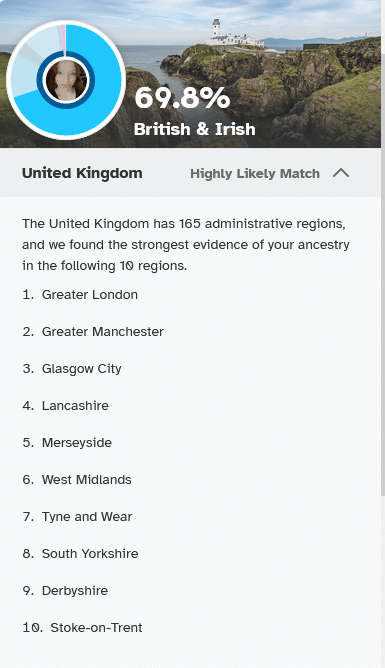The image features a gray background with a profile picture of a girl prominently displayed within a circular frame, which is highlighted with blue and gray accents. The text indicates a genetic ancestry composition showing that she is 69.8% British and Irish, with a highly likely match to the United Kingdom. The analysis identifies her strongest ancestral connections across 10 specific regions within the UK, which include:

1. Greater London
2. Greater Manchester
3. Glasgow City
4. Lincolnshire
5. Merseyside
6. West Midlands
7. Tyne and Wear
8. South Yorkshire
9. Derbyshire
10. Stoke-on-Trent

Additionally, it notes that the United Kingdom comprises 165 administrative regions.